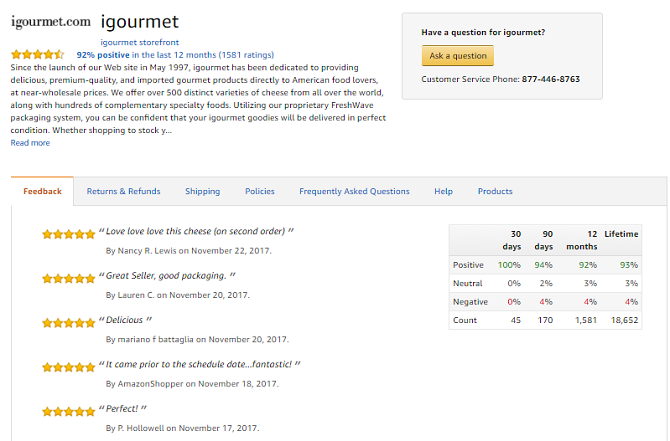The image depicts a review page for iGourmet.com, with an entirely white background and predominantly black lettering. In the top left corner, "iGourmet.com" appears in small black letters, while a larger "iGourmet" is placed to the right. Below this, the text "iGourmet Storefront" is displayed in blue letters.

This review page showcases a store performance summary: on the left side, there are four and a half yellow stars out of five, with a note stating "92% positive in the last 12 months" and "1,581 ratings," all presented in blue letters. Additional review information is provided underneath.

On the right side of the page, there is a gray square box. Inside, in black letters, it reads "Have a question for iGourmet?" Below this, a yellow banner within the gray box invites users to "Ask a question" in clickable black letters. The box also contains a customer service phone number, "877-466-8763," written in black letters.

Further down, individual ratings are shown. Five entries, each with five yellow stars, signify excellent reviews. On the right side of this section, another box summarizes the ratings over various time frames: the past 30 days, 90 days, 12 months, and the lifetime of the iGourmet storefront.